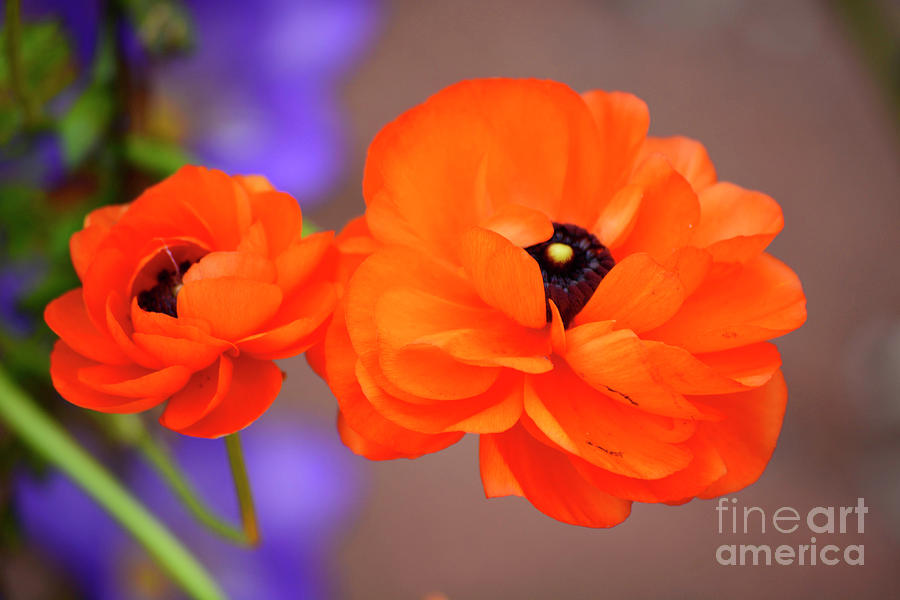This is an artistic, close-up photograph of two vibrant orange poppy flowers, captured in exquisite detail. The flower on the left is a smaller, mostly closed bud, while the one on the right is fully open, revealing a nearly black center with a distinct yellow dot in the middle. The bright green stems of the poppies prominently extend to the left back side of the photo. The background is intentionally blurred, transitioning from a purplish-blue hue on the left to a light gray on the right, with some leaves faintly discernible amidst the blur. In the bottom right corner, the image features a stylized, transparent gray watermark that reads "Fine Art America," indicating potential digital editing to enhance its artistic quality.